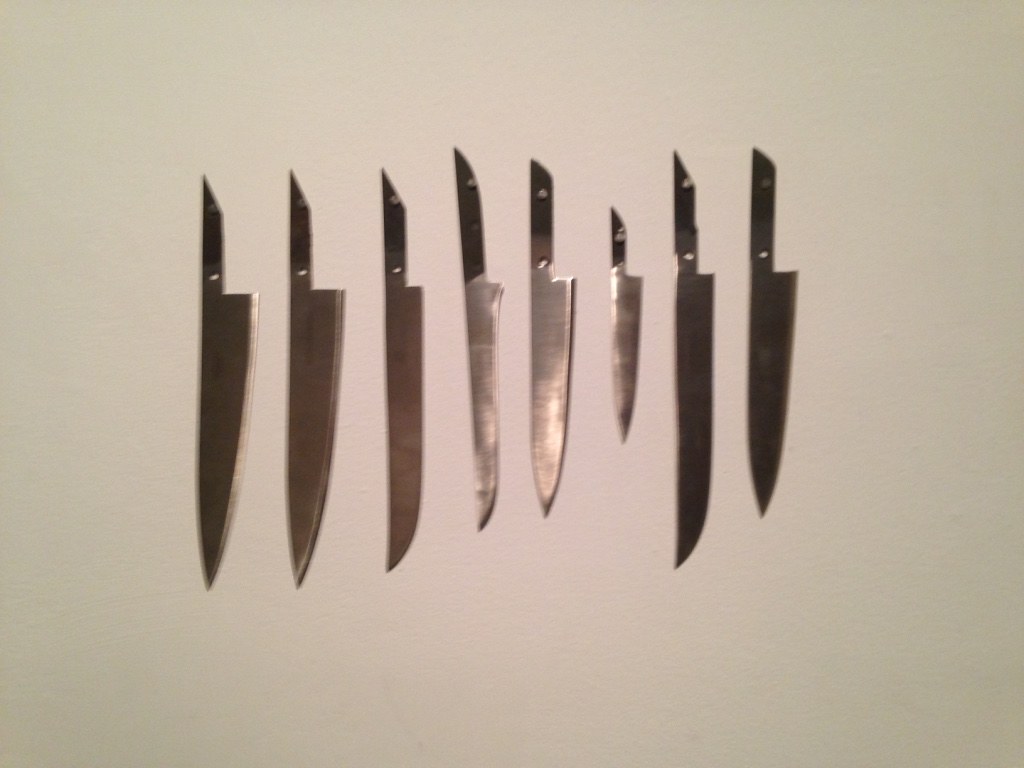This image showcases an overhead view of eight knife blanks, meticulously arranged side-by-side against a white background. These knife blanks vary in shape and length, indicating they will be transformed into various types of cutlery, likely used for kitchen purposes such as cutting meat, vegetables, or fruit. The blades, partially polished and ground, come to fine points and display a preliminary edge, though none are fully sharpened. Each blade has an attachment point, visible as drilled holes in the metal tangs, intended to be fitted into future handles. Despite one blank appearing relatively small, possibly intended as a steak knife, the rest are larger, thick blades suited for professional kitchen tasks. The blanks exhibit the style of Japanese knife craftsmanship, with the potential to be finished into beautiful, high-quality cutlery.